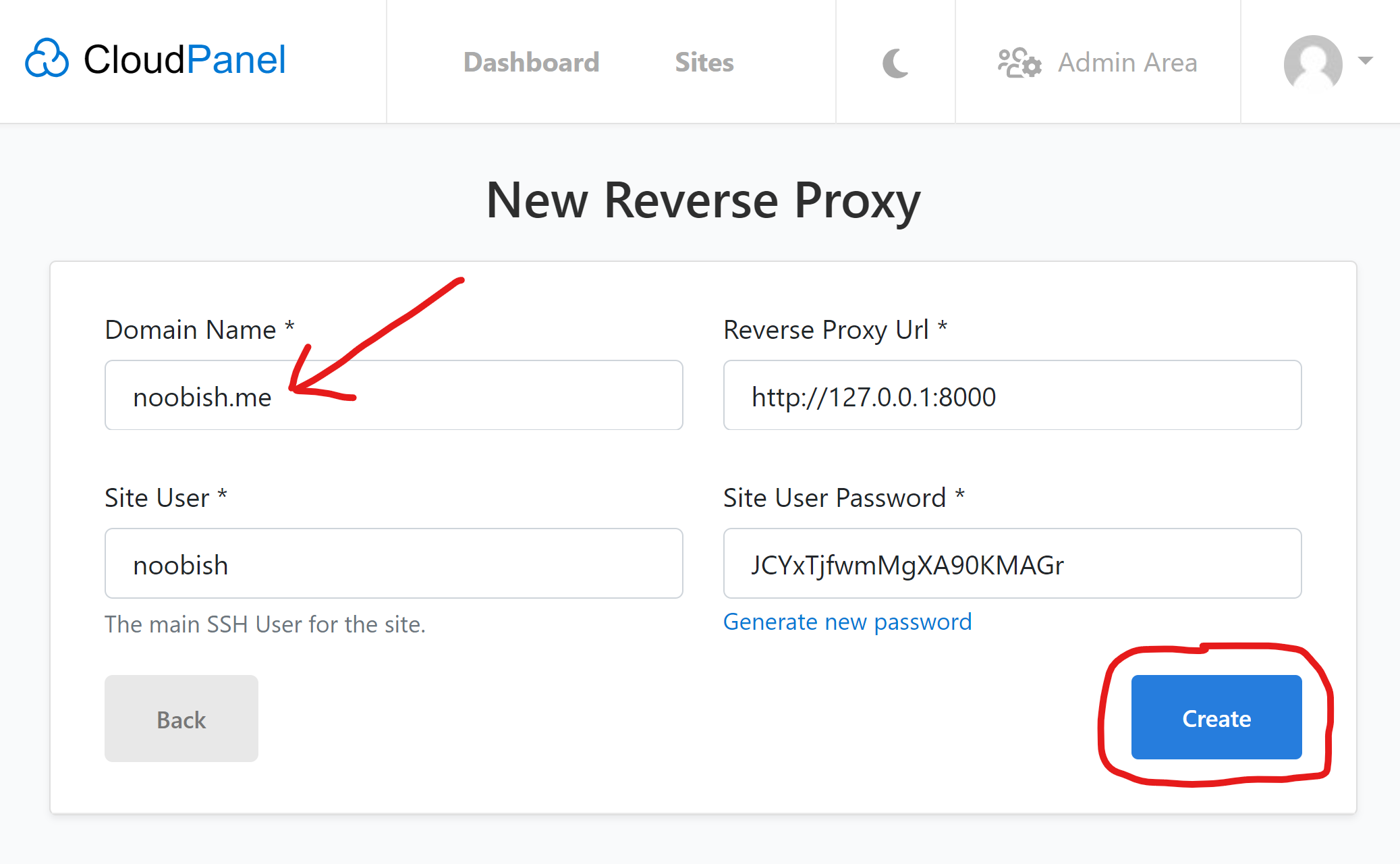The image appears to be a screenshot of a web-based interface, likely related to managing cloud services. The background is predominantly white, typical of a computer or smartphone screen.

Starting from the top left, the screen features a blue-outlined cloud icon followed by the text "Cloud Panel" in black and blue, respectively. Below this header, there is a light gray divider. The following sections are organized in a vertical list separated by light gray lines: 

- "Dashboard" in dark gray
- "Sites" in dark gray
- A filled-in crescent moon icon in gray
- An icon depicting two people with a settings gear, labeled "Admin Area"
- A profile picture icon with a downward arrow indicating a dropdown menu

The main content area beneath these headers is a slightly darker shade of gray. At the center, bold black text reads "New Reverse Proxy." Below this title is a white input box labeled "Domain Name*" with "newbush.me" typed in and a red arrow pointing at it. Another input box follows, labeled "Site User*" with "newbush" filled in, accompanied by a note that says "The main SSH user for the site." 

Next, there is a grayed-out "Back" button. The form continues with a "Reverse Proxy URL*" field displaying HTTP information. Another "Site User*" field appears with an associated password input and a link in blue that reads "Generate New Password." 

At the bottom of the form, a blue button labeled "Create" in white text is prominently circled in red, indicating a primary action button for the user.